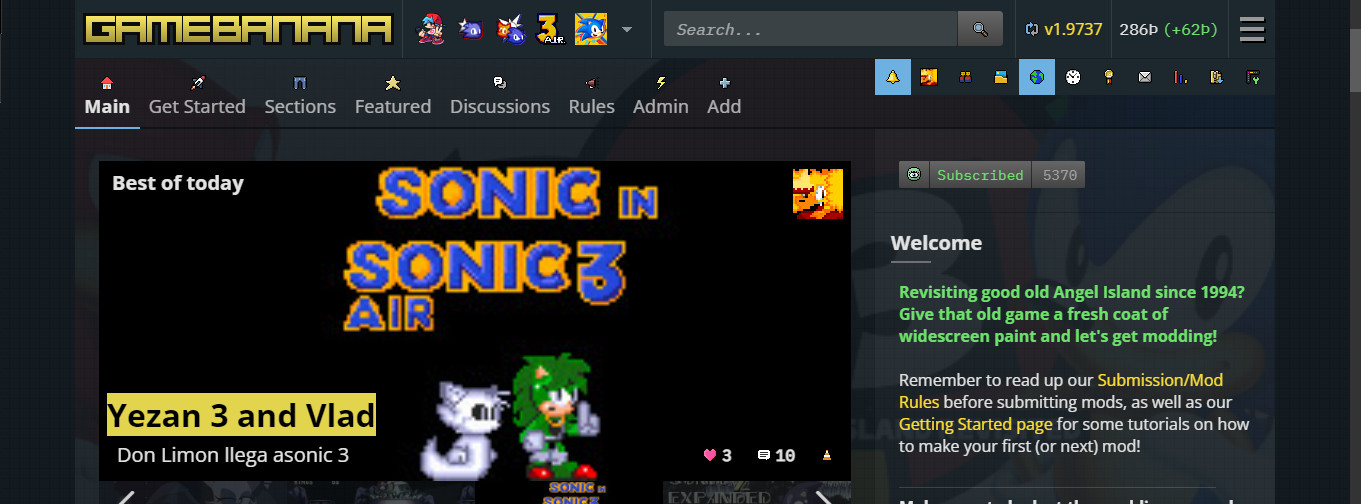This is a screenshot taken from the gaming website "Game Banana." The background of the webpage is predominantly black, creating a striking contrast against the various colorful elements. In the upper left-hand corner, the site’s name "Game Banana" is prominently displayed. Below the header, there are various icons representing different games. At the top of the webpage, five clickable icons are visible, although more are likely accessible via additional navigation.

A search bar labeled "search..." is present, allowing users to search the site. The page version "191.9737" is noted, along with two strings of numbers, "286B" and "62B," whose context is not immediately clear. On the left side of the screen, a vertical navigation menu lists options including "Main," "Get Started," "Sections," "Featured," "Discussions," "Rules," "Admin," and "Add."

In the "Best of Today" section, a highlighted feature is "Sonic 3 Air" by Yazan 3 and Vlad, with the description "Don Lamon Illiga a Sonic 3." This section also includes an engaging welcome area adorned with images of Sonic the Hedgehog, adding a vibrant and iconic touch to the page.